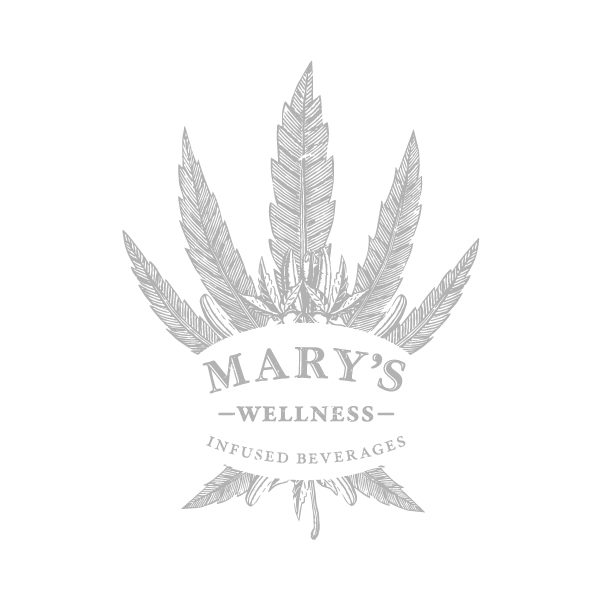The logo appears in black and white against a light gray background, featuring an intricate plant design with numerous fronds similar to a fern. In the center of the logo, a white oval cutout showcases the business name in three distinct lines of text. The largest text reads "Mary's" in an old-timey font, with an emphasis on size. Beneath it, "Wellness" is displayed in all caps with a dash on each side, and finally, the smallest text, "infused beverages," appears in a different, less bold font. The plant design features various elements, including three small leaves at the center and five larger fronds arching upward around the text. Additional smaller fronds appear both near the logo’s center and at the bottom, adding to the intricate, layered botanical theme.